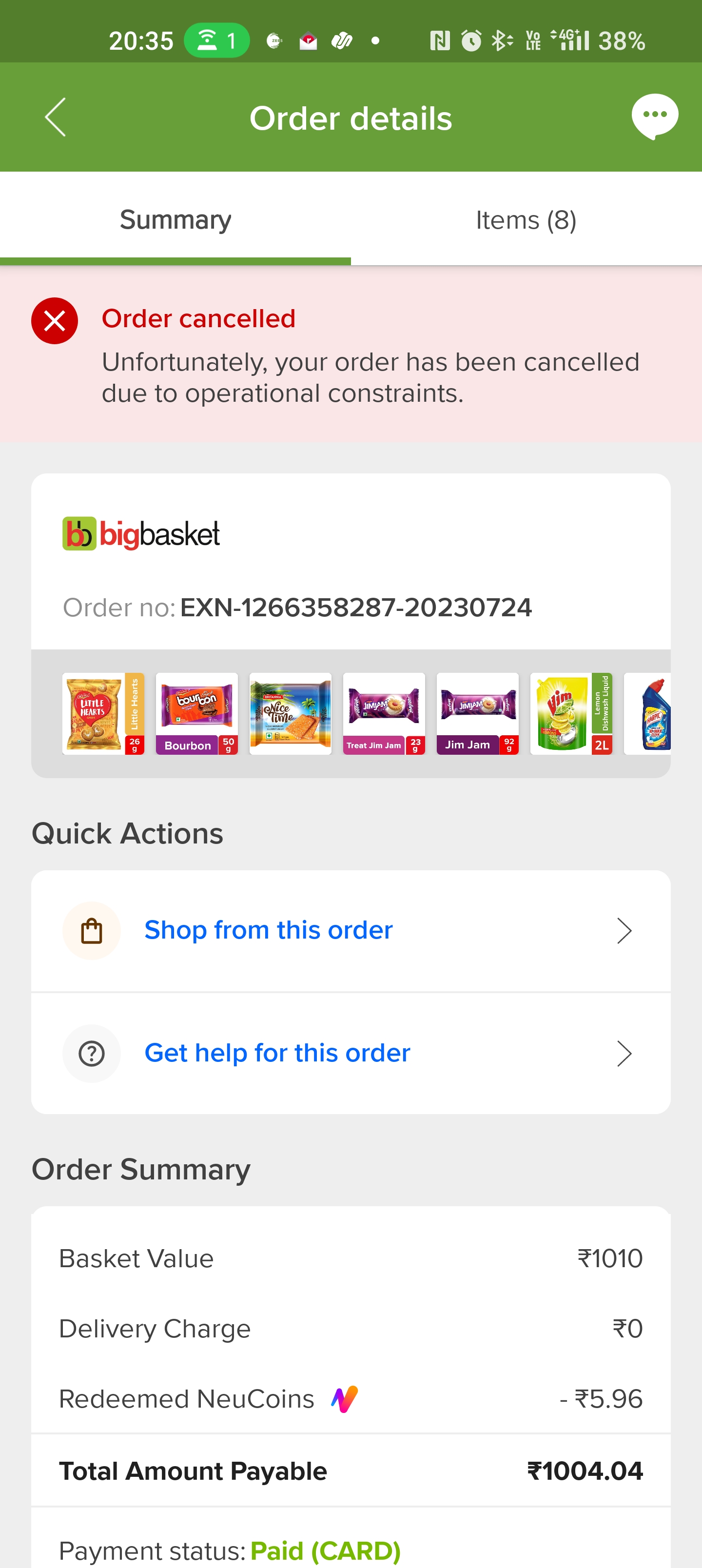This image, captured from a smartphone device, is presented vertically. At the very top, the screen displays a dark green rectangular strip followed by a lighter green rectangle. The time “20:35” is shown in military format, accompanied by various icons including a green symbol and different white icons to the top right, such as a clock and Bluetooth status, with a battery life indicator showing 38%.

Below this, a green rectangle features the heading "Order Details" in white. To the right of this heading, a chat icon with three dots is visible. In black text, "Submarine" is displayed, followed by "Items (8)" indicating the number of items in the order.

Unfortunately, a red box with darker red font indicates that the order was canceled, showing a red circle with a white X. The text reads: "Unfortunately, your order has been canceled due to operational constraints."

Beneath this, a white box shows the vendor “Big Basket” along with the order number. The section below features icons representing the different items ordered, offering quick actions such as "Shop from this order" and "Get help for this order," both highlighted in blue.

The order summary includes details such as:
- Basket value: $1,010
- Delivery charge: $0
- Redeemed new coins: $5.96
- Total amount payable: $1,004.04
- Payment status: "Paid by card" in green text.